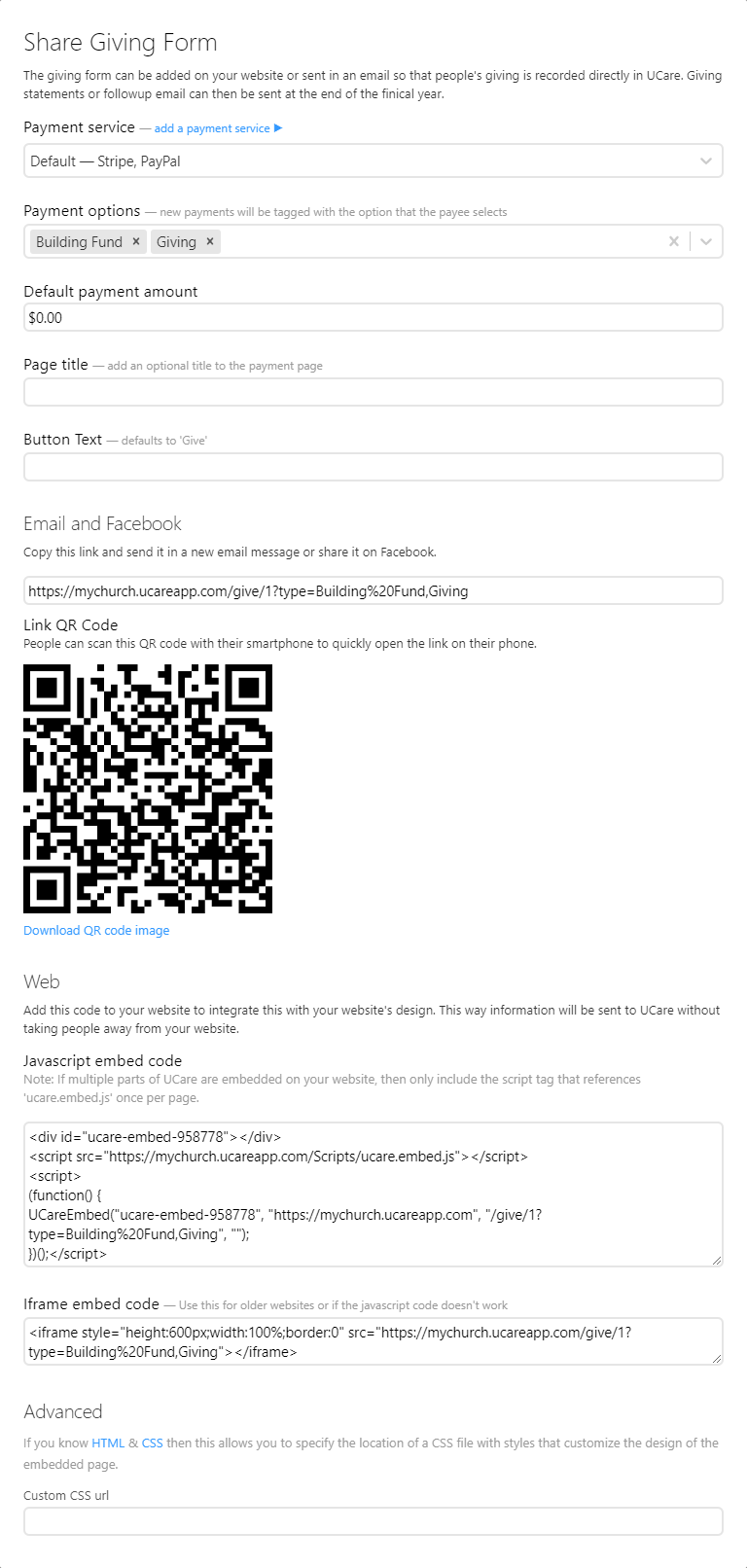A computer screen displaying a detailed form titled "Share Giving Form" at the top. The form features a white background with black text and a small paragraph beneath the title. A drop-down menu allows users to select options, followed by three blank input boxes for additional information. Below these, options for email and Facebook are listed, accompanied by a small amount of writing. A rectangular field appears to contain a web address, followed by a "Linker Code" and a brief sentence. There's a square QR code available for scanning with a phone, and beneath it is some blue text followed by more black text. The form also includes another densely filled square section with a heading, a secondary rectangular information box, and an "Advanced" section with a sentence, part of which is in blue text. The bottom of the form includes an additional blank rectangular input field.